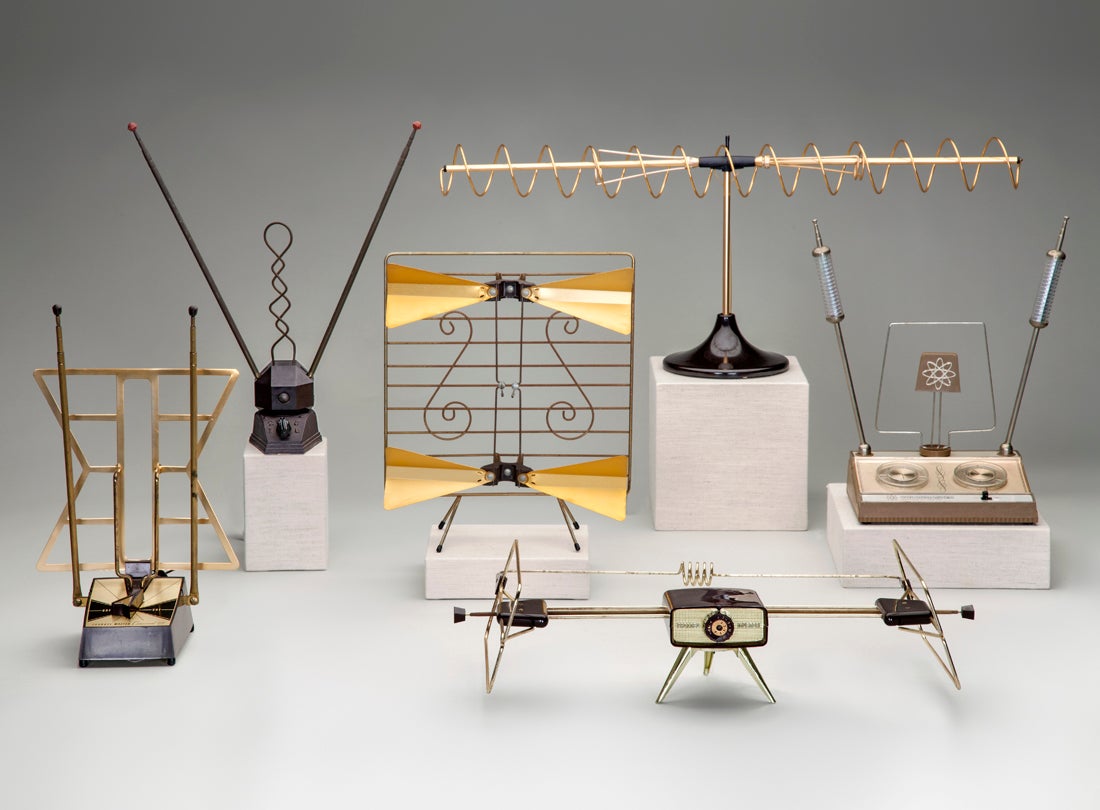The image displays a collection of six diverse antennae and various pieces of technological equipment positioned side-by-side on a flat, white surface, all against a white wall background. Each antenna has a unique design and is made up of silver, gold, and black components. On the far left, there's an antenna with prominent gold framing attached to a black box, featuring a diamond-shaped dial. To its right, there's a device resembling a black antenna on a white block, equipped with two long antennas extending to the left and right. Centrally located is a gold grid-like object adorned with solid gold, sideways triangles on the top and bottom, accompanied by a design that resembles a reversed 'S' and a normal 'S'. Adjacent to this is an antenna mounted on a white stand with silver legs ending in rubber black tips, showcasing a grill-like structure. Another piece, positioned centrally, features a tall silver pole wrapped with a gold wire, supported by a black base atop a larger white platform. The sixth antenna rests on a smaller white box, displaying a neutron symbol and two silver knobs, with square-like antennas protruding from each side. The image is well-lit, vividly colored, and clear, ensuring all the details of each piece of equipment are visible without any blurring or distortion.